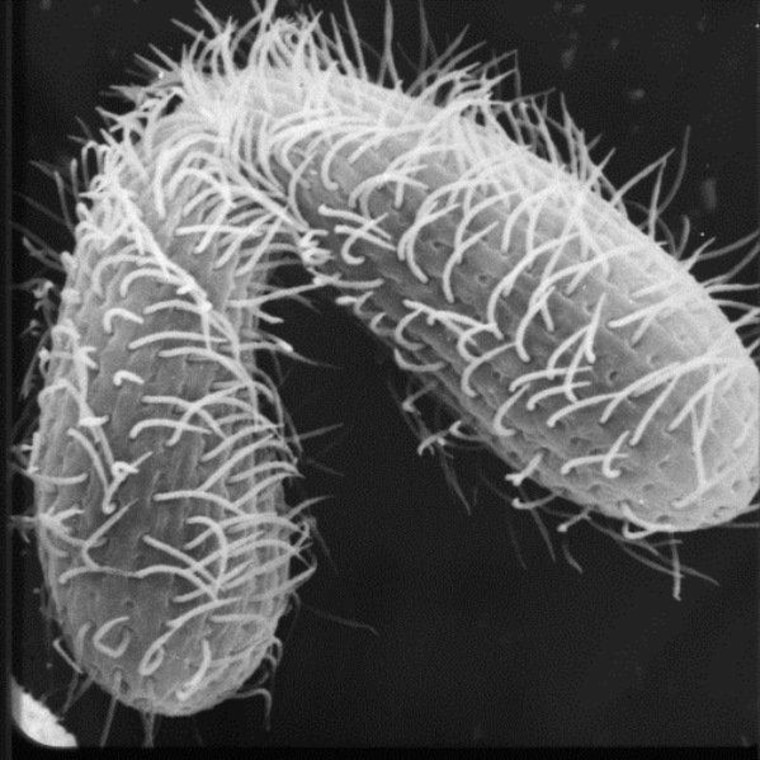This microscopic photograph captures a cactus-like object against a dark grey to black background. The primary structure is V-shaped, resembling an upside-down "V" or boomerang, with two lobes joined at a central bend. The left lobe is vertical, while the right lobe extends downward and to the right. The surface of the object is light grey with faint white ridges, suggesting a leather-like texture. Covering the entire structure are numerous fine, white tendril-like hairs, with a higher concentration at the bend. These hair follicles vary in thickness, with some being very fine and nearly transparent against the dark background. Additionally, in the bottom left corner of the image, there is a rough white triangular shape, adding an intriguing element to the frame.